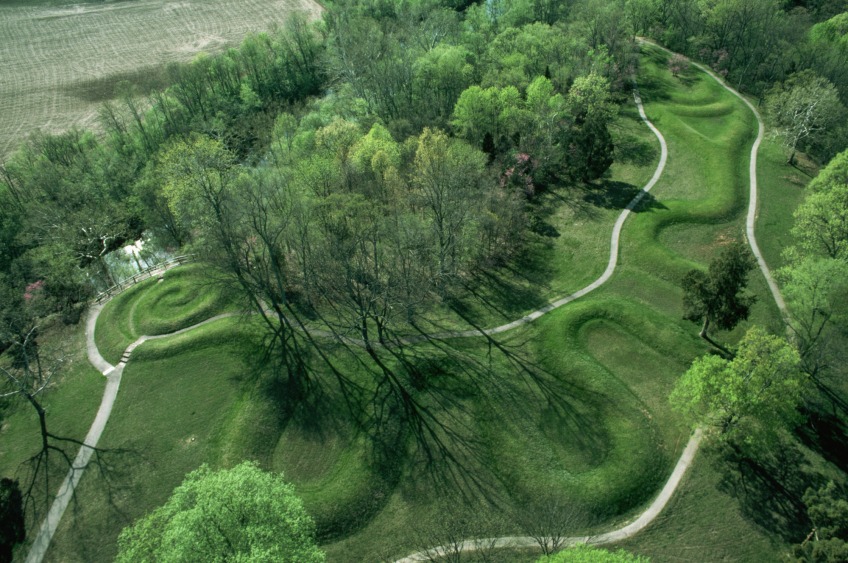The image is an aerial shot capturing an intricately manicured park and surrounding nature. The top part of the picture is dominated by a dense grove of tall, green trees. Below the trees, two parallel, white paths stretch across the scene, each featuring a mix of straight and slightly curved segments. Between these paths, grass and plants have been groomed into an elegant S-pattern. On the left side of the image, a field resembling a farmer's plot appears, hinting at agricultural activity. Additionally, a small pond can be seen, and various winding trails, possibly meant for walking or driving, weave through this meticulously maintained garden. The overall landscape blends natural greenery with man-made elements, evoking the image of a serene, forested park, potentially even a golf course, given its pristine condition.